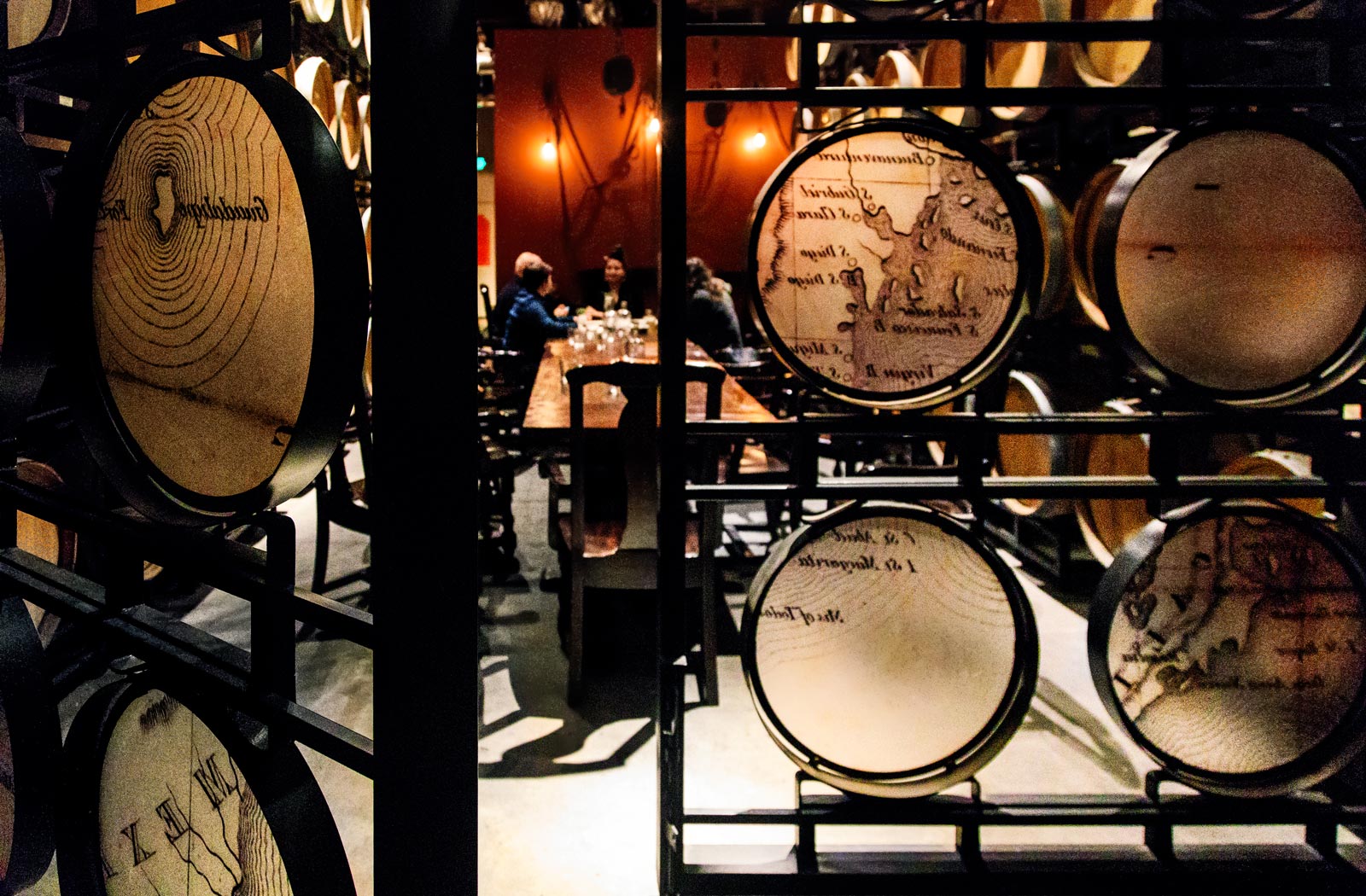The photograph depicts a dimly lit bar or dining area framed by intricate wrought iron dividers. These dividers form a grid pattern with circular frames, each displaying different items—some appearing to be maps and others resembling slices of tree trunks. Through the openings in the dividers, the scene within the room unfolds, revealing a long wooden table surrounded by chairs. Around the table, three or four people are engaged in conversation, with glasses and bottles scattered on the surface. The ambience is accentuated by walls painted in dark orange, illuminated by bright white lights that cast an orange glow, creating a warm, cozy atmosphere. Stepping into this scene feels like entering a space defined by a blend of rustic charm and intricate decor, where every element contributes to a rich visual experience.